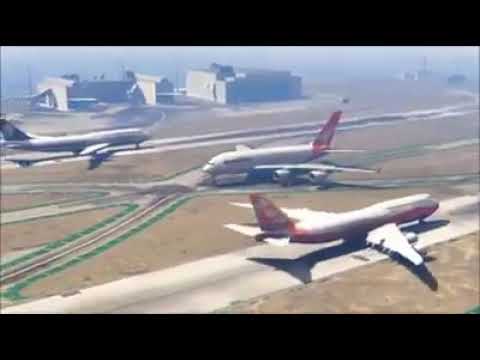The image depicts an airfield captured from an elevated perspective, approximately 50 to 75 feet above the ground. It is unclear whether the photograph is from an actual camera or a screenshot from a video game, as the overall quality appears slightly blurry and hazy, giving an aged or cloudy appearance. The image is framed with black borders at the top and bottom and is wider than it is tall.

In the foreground, there is a large jumbo airplane on a cream-colored runway with distinct black tiger stripes. This airplane is oriented towards the right side of the image, featuring a white upper fuselage, a red lower section, and a red tail. Its long wings extend beyond the edges of the runway, and an engine is visible underneath one of the wings on the right side.

Centrally located is another jumbo airplane, also on a runway. This airplane is facing to the left and has a white body with red decals near the cabin area. Visible are two engines mounted beneath its wings and a red tail.

Further to the left in the image, a third airplane is positioned on a runway, pointing towards the upper right of the frame. This airplane has a white top, a blue stripe along its body, and appears either about to land or take off.

In the background, two buildings are visible: one solid structure with cream-colored walls on the right and another building with cream-colored walls and an open center on the left. The distant scenery is shrouded in a haze, adding to the image's indistinct quality.